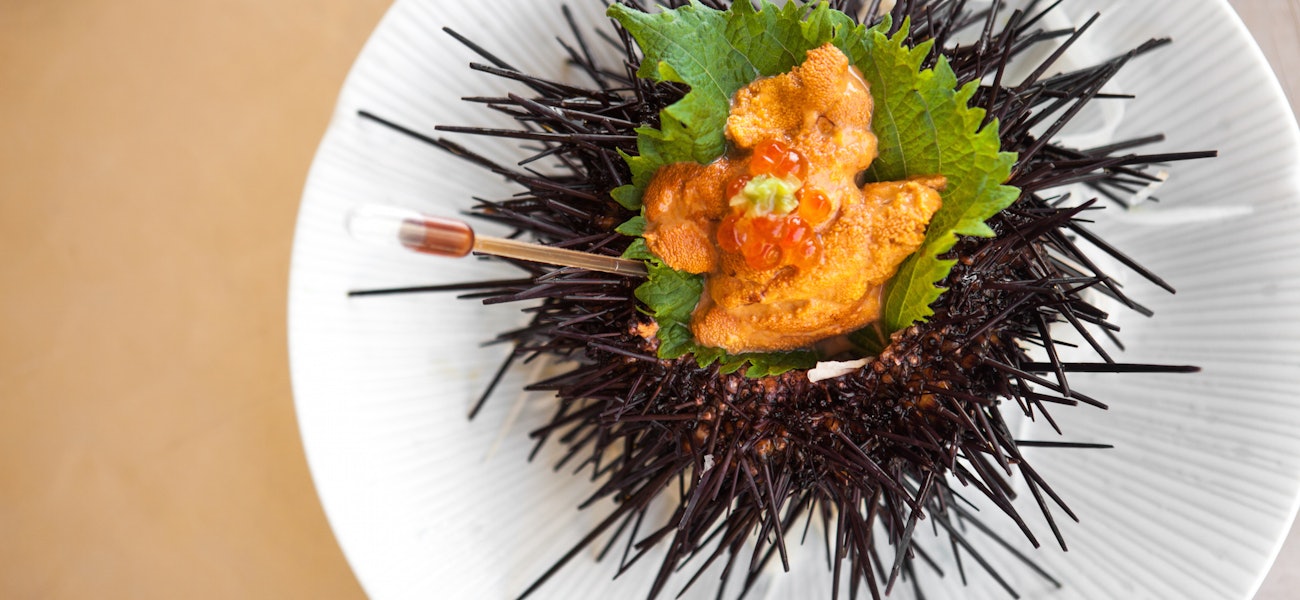The image depicts a meticulously arranged dish at what appears to be a five-star restaurant. The setting shows a white plate adorned with fine ridge lines radiating from its center, placed against a background that is predominantly tan with hints of gray. At the heart of the plate lies a dark brown sea urchin, displayed upside down with its spiky spines prominently visible. Nestled within the sea urchin are several green leaves, likely part of a salad mix. Topping this are fish eggs or roe, colored in shades of orange and red, alongside a yellowy-brown and light orange mixture, artistically arranged. A golden spoon or a seafood fork handle protrudes from the left side, completing the intricate presentation of this gourmet sea urchin dish.